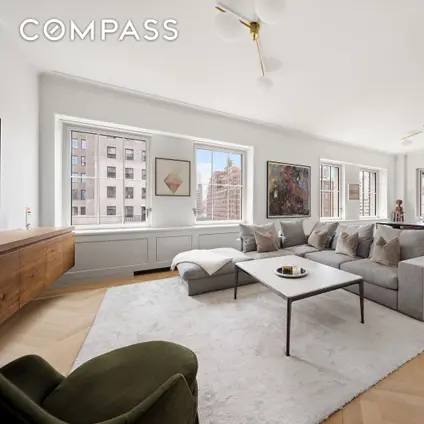The image depicts the interior of a well-lit room. The word "campus" is written in white text in the top left corner. The ceiling is painted white and features a central gold ceiling fan adorned with white light bulbs on each blade. The walls are also white, complementing the white-framed windows. On the left side of the room, there is a brown, wall-mounted cabinet. 

Dominating the center of the room is a gray carpet, upon which sits a white table with black legs. On this table is a plate. To the right of the table is a gray L-shaped couch, complete with matching gray cushions. Directly above the couch, centered on the wall, is a picture frame that features a black and white image. Another picture frame to the right displays flowers in pink, green, and brown hues.

The room's floor outside of the carpet area is brown. In the bottom left corner, there is a single green couch with darker shades. Through the windows, one can see a tall building to the left and a slightly maroon-colored building through the second window. Lastly, the area below the wall-mounted cabinet reveals a continuation of the brown floor.